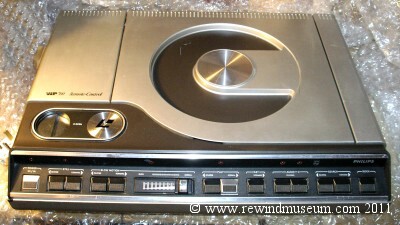This is a color photograph of a vintage piece of audio equipment, likely a CD player given its design. The equipment features a flat, rectangular, polished silver cabinet with a lift-up lid for inserting discs. The front panel is adorned with more than ten buttons, predominantly black, each labeled with various functions that are too small to read in this low-resolution image. A pair of white knobs and several black knobs and flip switches, including what appears to be a number counter, hint at its complex functionality. Immaculately preserved, the device displays a noticeable watermark in the bottom right corner, reading "www.rewindmuseum.com 2011," indicating its inclusion as an artifact in the Rewind Museum collection.